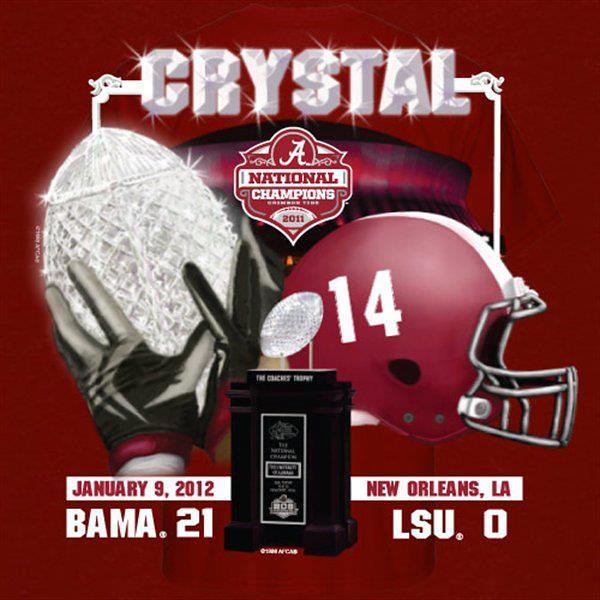This graphic design poster commemorates the 2011 National Championship game between Alabama and LSU. Dominating the composition, the top of the poster features the word "CRYSTAL" in sophisticated, beveled white letters with sparkles and lens flare effects. Below, the iconic Alabama football helmet, primarily red with a white stripe down the center and sporting the number 14, is turned to the side, showcasing its face mask and shield logo with the emblematic white 'A'. 

At the center, a pair of black gloves with dark gray stripes and red and white accents around the wrists hold up a dazzling crystal football, symbolizing the National Championship trophy. A closer look reveals another crystal football trophy set on a sleek black pedestal, located in front of the helmet with an indistinct plaque.

The bottom portion details the game's essentials: on the left, a white rectangle states "January 9, 2012," while the right rectangle indicates "New Orleans, LA," the venue. Beneath this, the score is prominently displayed in bold white and red text: "Bama 21, LSU 0" against a rich maroon background. Moreover, the phrase "National Champions 2011" is elegantly inscribed within a white rectangle, completing this celebratory tribute. The backdrop subtly integrates an illustration or photograph of the stadium, enriching the historic and victorious narrative depicted in the design.